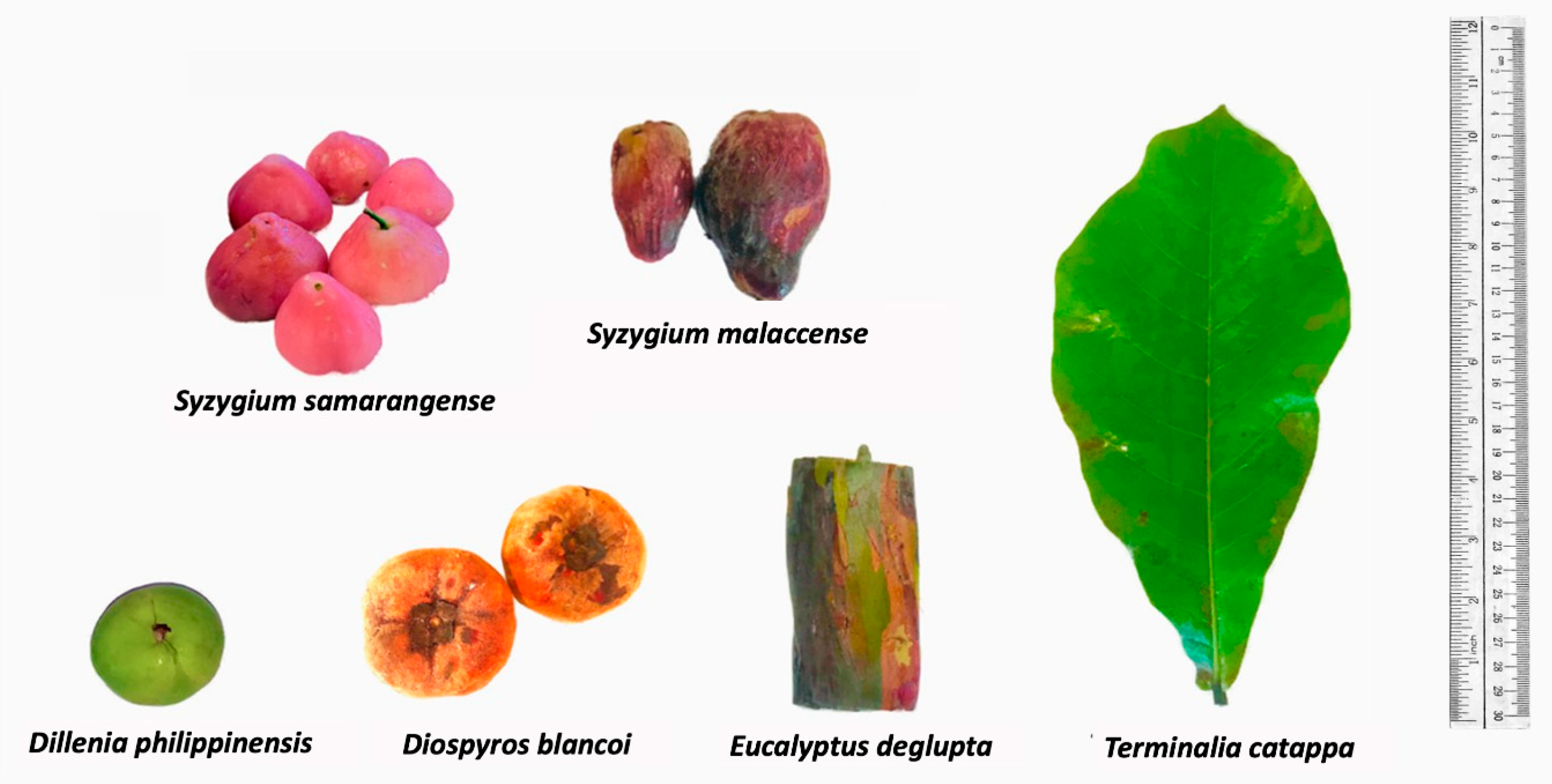The image depicts a detailed exhibit showcasing various fruits, leaves, and plant parts, each labeled with scientific names. On the far right, a gray vertical ruler with measurements serves to indicate the size of the specimens. To the immediate left of the ruler is a large green leaf labeled "Terminalia catulpa." Adjacent to the leaf is a piece of bark labeled "Eucalyptus deglupta." Moving left, there are two orange fruits labeled "Diospyros blancoi," and further left is a single green bulbous fruit labeled "Dillenia philippinensis." In the top left corner, a cluster of pink fruits is labeled "Syzygium samarangense," while next to it, a small cluster of fruits labeled "Syzygium malaccense" can be seen. All items are presented against a gray background, giving a clear and organized display suitable for educational purposes.